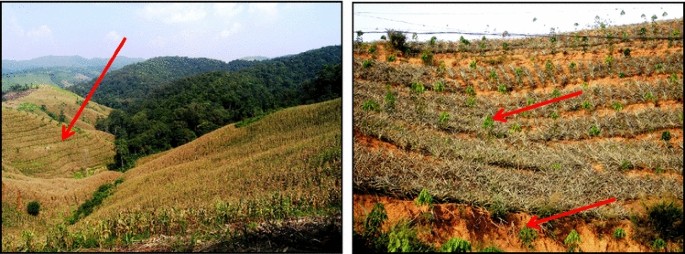The set of two color photographs features a detailed, hilly landscape scene on the left and a zoomed-in view of part of this landscape on the right. The left image captures rolling hills covered with tan, dry grass and scattered green patches, transitioning into denser greenery of trees in the middle. Beyond, successive layers of hills, from green-gray to blue-gray, culminate in a light blue sky accented with numerous white clouds. A prominent red arrow points to a furrowed area on one of the hills.

The right image provides a close-up of the aforementioned furrowed hill, showcasing the ground with exposed brown dirt and dry, dead vegetation. Two red arrows in this image highlight parts of the landscape: one points to a small green plant emerging from the barren earth, and the other targets another area of the exposed ground. Despite the agricultural appearance, the vegetation, predominantly dead grass and weeds, seems sparse and struggling, adding a poignant touch to the scene.